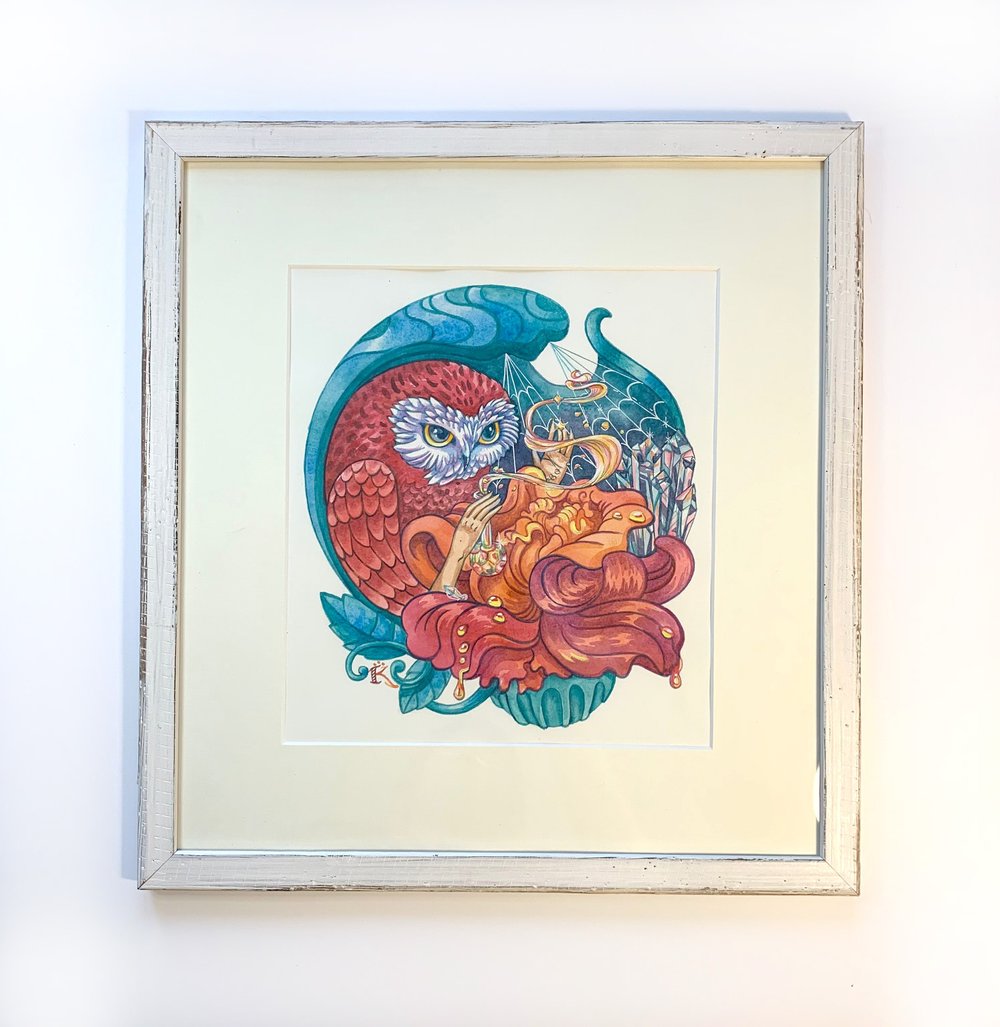The image showcases a vibrant piece of abstract art mounted on a white wall, housed within a white wooden frame. Inside the frame, the artwork sits on a milky-colored platform and features an inner white border surrounding the main painting. The central figure in the painting is a red owl with a white face, a yellow beak, greenish eyes, and human-like hands raised upwards. The owl appears to be enveloped in a green background and is adorned with what resembles rose petals and a container emitting gas. To the far right, the scene includes a cityscape or clusters of crystals and cobwebs hanging from the top. The painting is brightly colored and intricately detailed, with the initial "R" in the lower left corner, presumably indicating the artist's signature. The overall image is clear, well-lit with natural light, and draws attention to the surreal and mystical elements within the artwork.